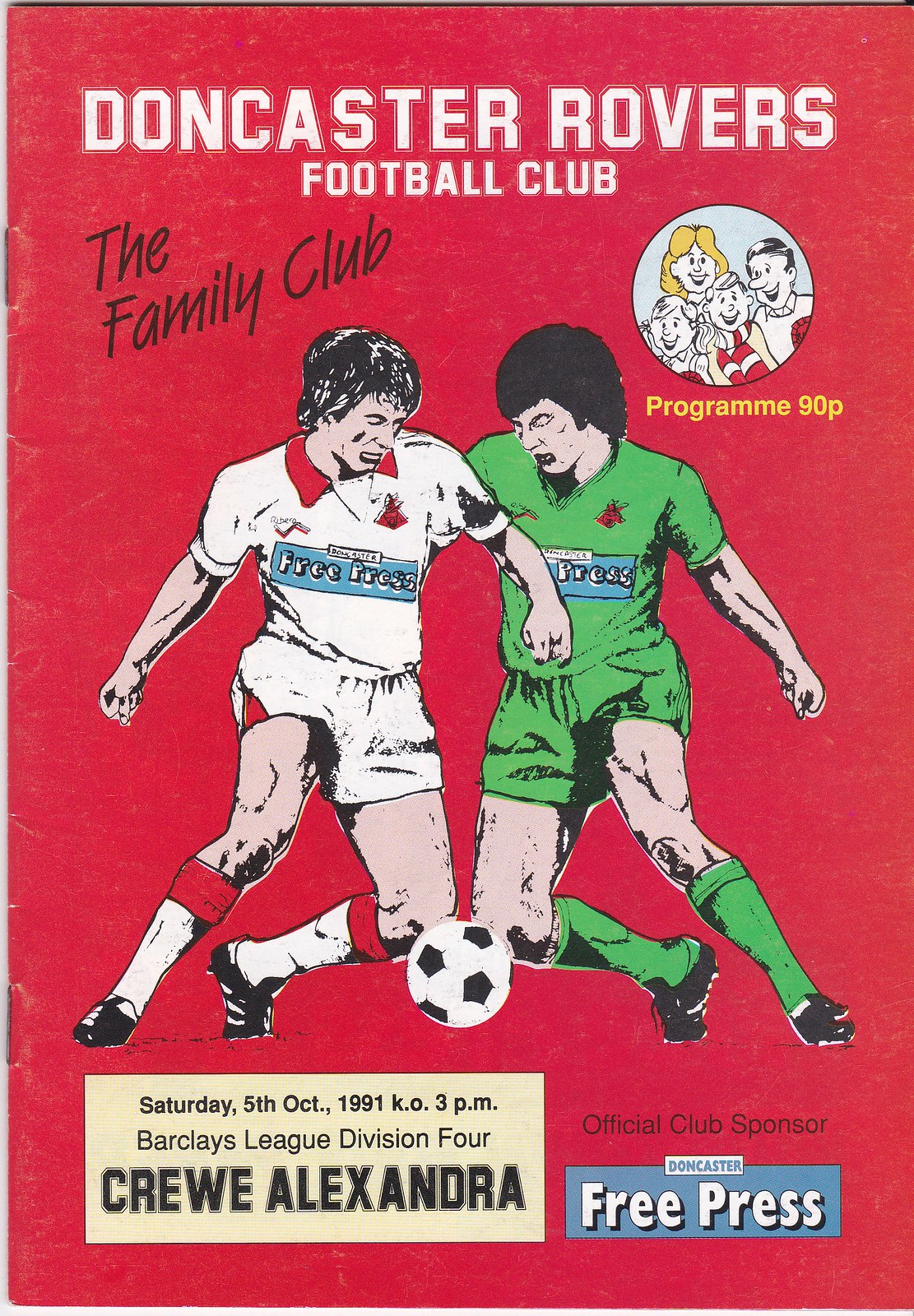The front cover of the Doncaster Rovers Football Club program for the October 5th, 1991 match against Crewe Alexandra showcases a vivid scene designed to emphasize the club's family-friendly atmosphere. Priced at 90 pence, this rectangular booklet features a predominantly red background with a striking depiction of two soccer players vying for a classic black-and-white soccer ball. The player on the left dons a white uniform with red accents, including red stripes on his socks and collar, and he has shaggy black hair. The opposing player, dressed in a green jersey, shorts, and socks, also has black hair. Above the action, a cartoon drawing of a family reinforces the club's family-oriented branding. The top of the program reads "Doncaster Rovers Football Club, The Family Club," and the bottom provides detailed match information: "Saturday 5th October 1991, 3 p.m., Barclays League Division 4, Crewe Alexandra." The official club sponsor is prominently noted as the Doncaster Free Press.